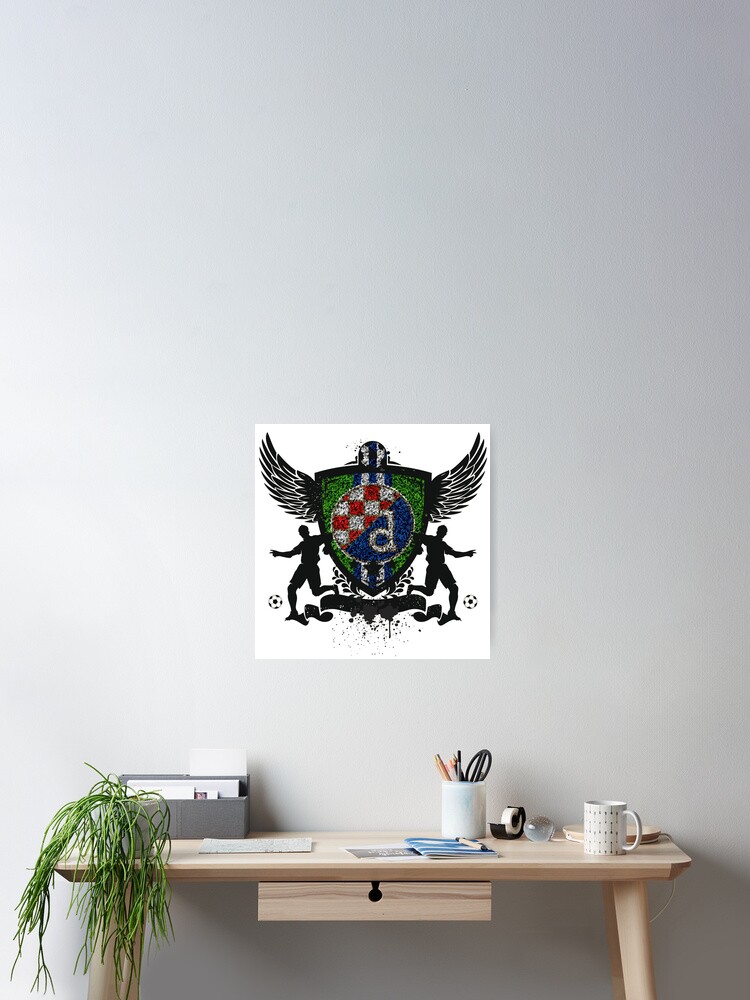The image depicts a modern interior showcasing a pale wood-colored desk with four legs and a central drawer featuring a keyhole opening. On the desk, there are various items including a white mug, a white container holding pencils and scissors, a black tape dispenser, scattered papers and booklets, a gray male organizer, and a green plant. Positioned on the edge of the desk is a sleek, white long-necked lamp with an adjustable arm, clamped on the right side, forming an upside-down L shape. The background wall is light gray, creating a neutral backdrop for a prominently displayed shield emblem. The emblem features a crest divided into two halves: one side with red and white checkers and the other side blue with a letter "D." Adorning the emblem are black wings and silhouettes of two soccer players in action, suggesting a logo for a football or soccer team. The overall setting gives off a clean, organized, and modern feel, similar to an IKEA advertisement.